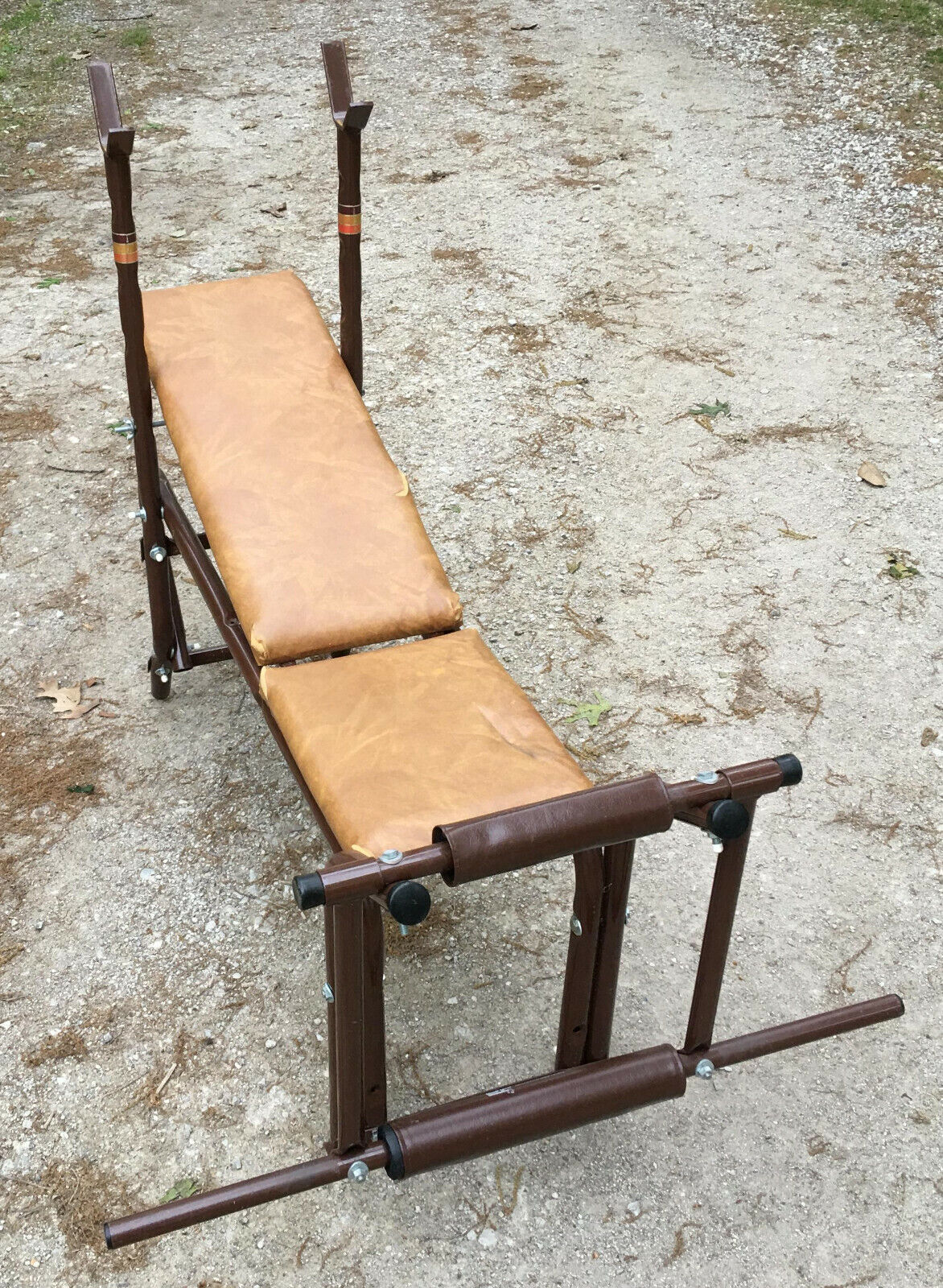The photograph captures an old, outdoor weightlifting bench positioned on a predominantly gravelly and rocky surface, with sparse patches of green grass visible in the background. This vertically rectangular image, taken during the daytime using natural light, focuses on the well-worn bench press. The bench features an inclined design with a small square seat and a longer rectangular backrest, both covered in light brown faux leather or vinyl, showing signs of age with visible tears. The metallic frame of the bench, including the supportive bars and leg extension equipment, is a dark brown color. At the end where the lifter's head would be, two upright bars extend upwards, ending in holders designed for a barbell, though no barbell is currently present. Additionally, at the foot of the bench, there is a leg press attachment with dark padding reminiscent of old bicycle handlebars, indicating a dual-purpose functionality for both upper and lower body exercises.